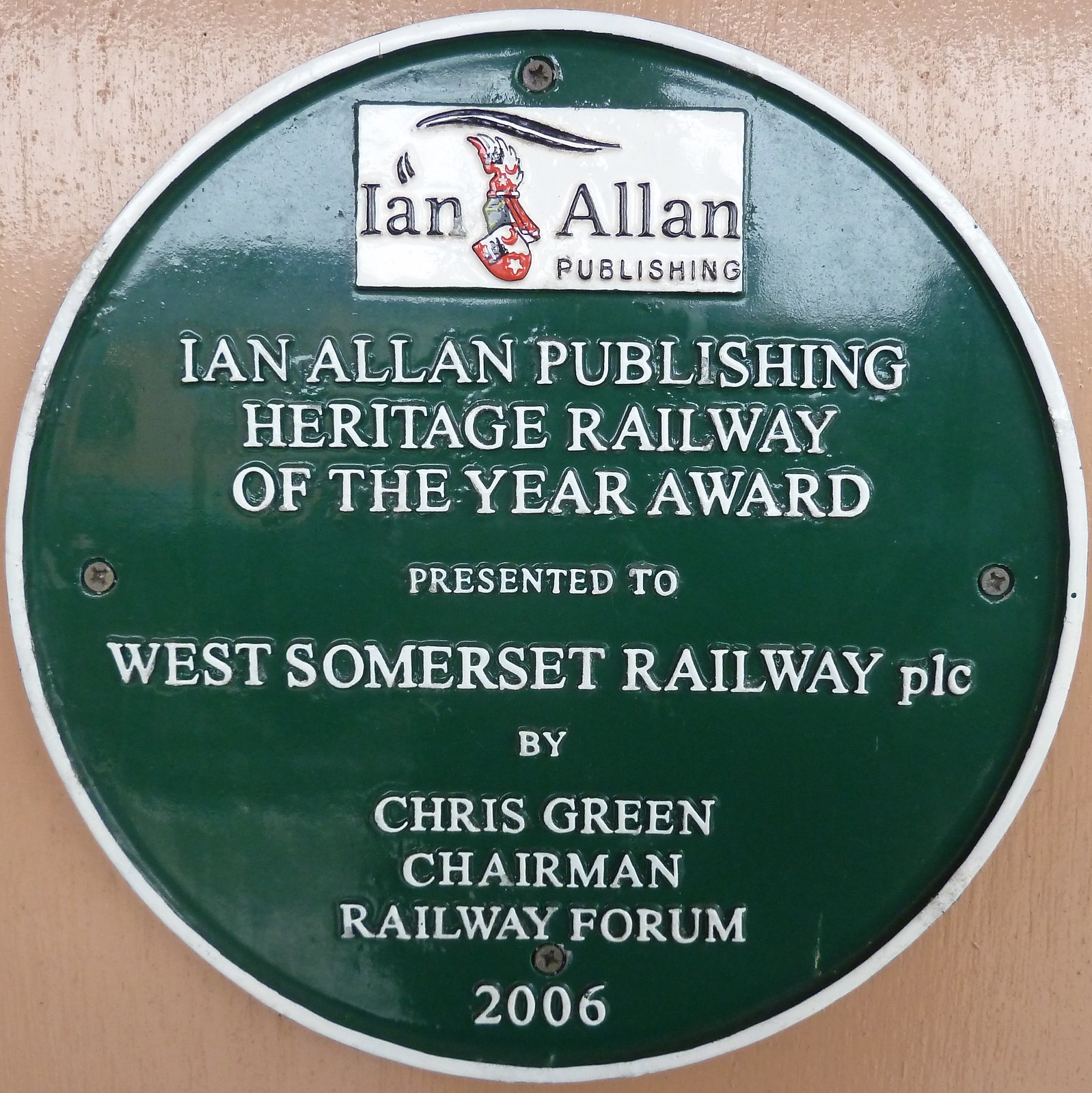This image depicts a close-up of a green circular metal plaque, affixed to a light brown wall. The plaque is encircled by a white outline. At the top of the plaque, inside a white rectangular box with black text, it reads "Ian Allen Publishing." Below this, in white font against the green background, it states "Ian Allen Publishing Heritage Railway of the Year Award." Further down, the text continues in white, reading "Presented to West Somerset Railway PLC by Chris Green, Chairman of the Railway Forum." The year "2006" is positioned at the very bottom of the plaque. The entire inscription is consistently in white font. There are four screws visible, securing the plaque: one at the top, one at the bottom, and one on each side.